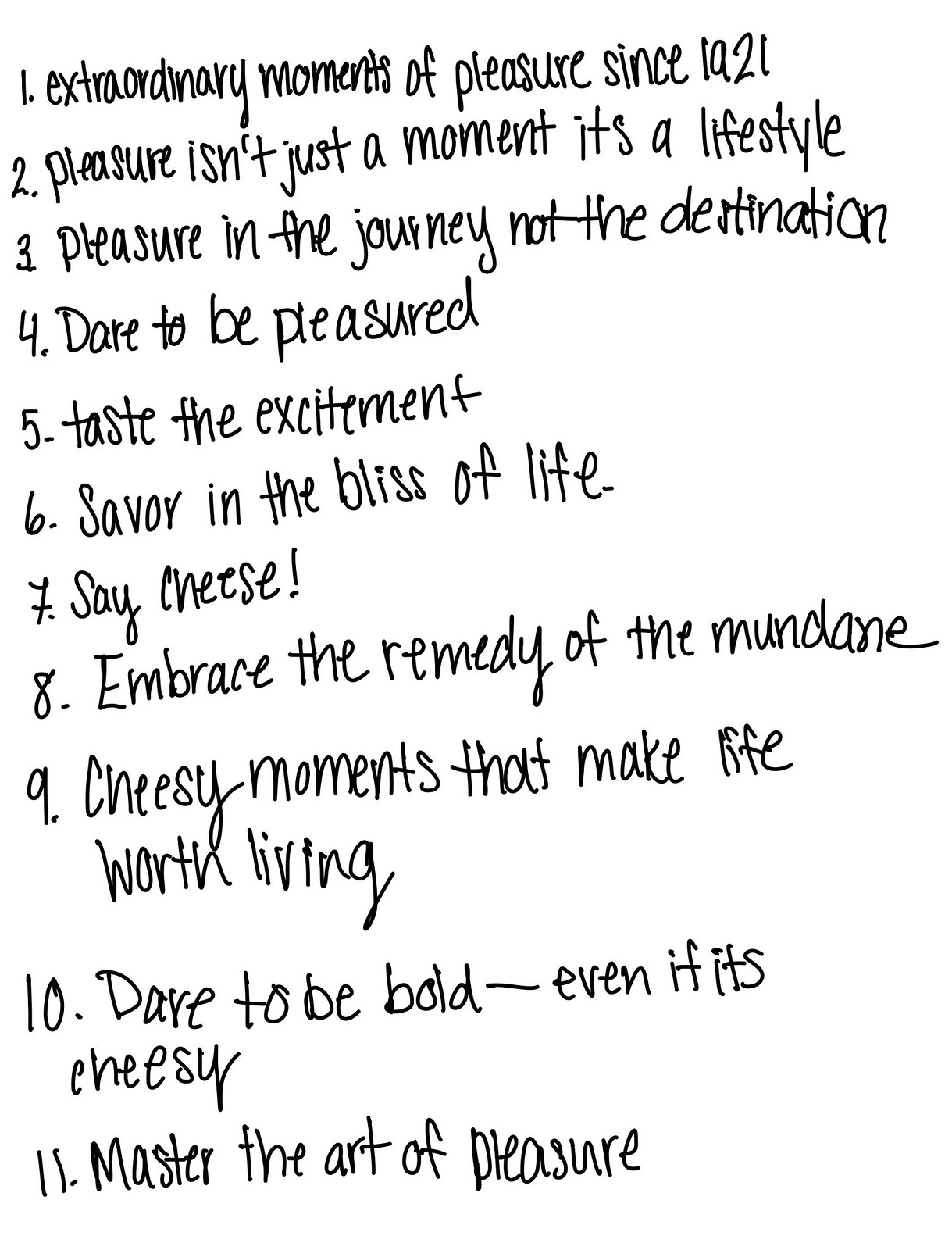This handwritten list, penned in curvy and informal black ink, appears on a white background, detailing a progressive series of numbered statements from 1 to 11. Each phrase emphasizes the theme of pleasure and integrates the concept of "cheesy moments" as a positive twist. The handwriting is distinct and varies slightly in size, with letters starting smaller at the top and enlarging as they descend. 

1. Extraordinary moments of pleasure since 1921.
2. Pleasure isn't just a moment, it's a lifestyle.
3. Pleasure in the journey, not the destination.
4. Dare to be pleasured.
5. Taste the excitement.
6. Savor in the bliss of life.
7. Say cheese!
8. Embrace the remedy of the mundane.
9. Cheesy moments that make life worth living.
10. Dare to be bold even if it's cheesy.
11. Master the art of pleasure.

Numbers 9 and 10 have unique line breaks, with "worth living" on a second line for 9 and "cheesy" on a second line for 10, indicating a rhythmic and personalized touch to the handwriting.